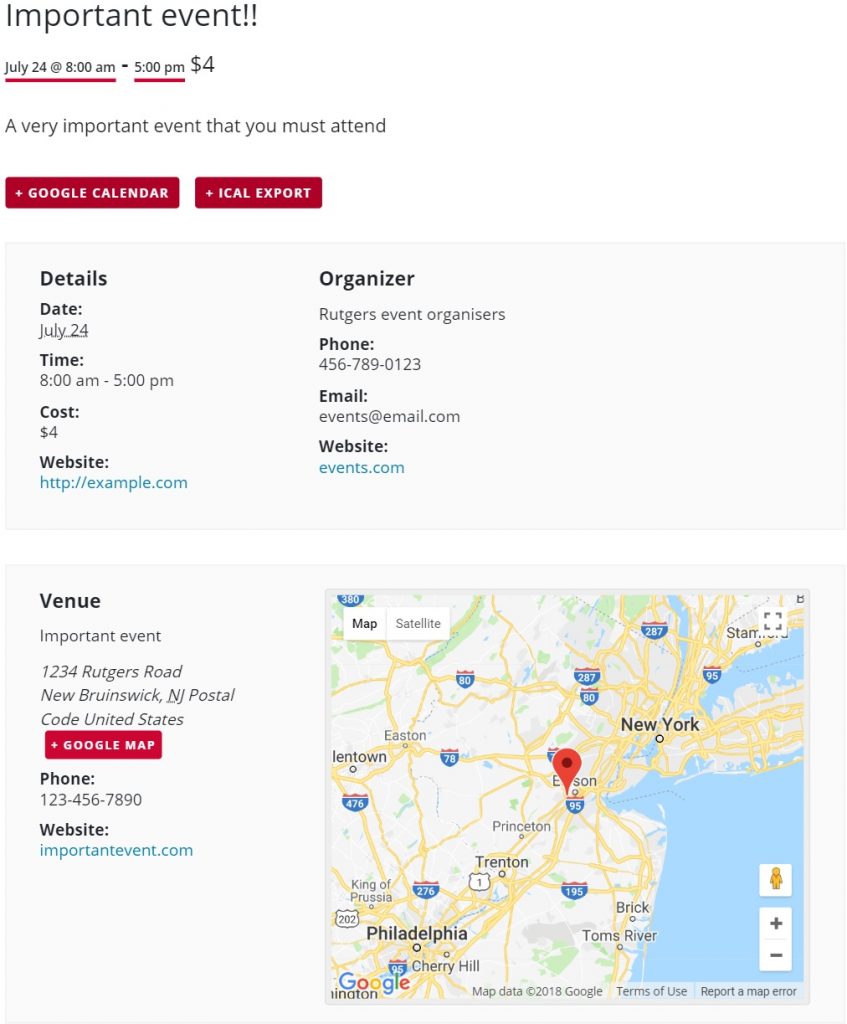**Important Event Announcement**

The vertical image is designed for viewing on a computer or smart device, featuring a white background.

At the very top, in bold black letters, the text "Important Event!!" is prominently displayed. Below this title, the event date and time are listed as "July 24th at 8 a.m." followed by a thick red underline, and "to 5 p.m." also underlined in red. The cost of the event, "$4," is clearly indicated. The text emphasizes the event's significance with the phrase "It's a very important event that you must attend."

Two red rectangular buttons are placed underneath this information. The buttons are labeled in white text: one says "Google Calendar" and the other says "iCal export."

Following these buttons, a gray rectangular box contains more detailed information in black text. It reads:

- Details
- Date: July 24th
- Time: 8 a.m. to 5 p.m.
- Cost: $4
- Website: (URL provided)
- Organizer: Rutgers Event Organizers
- Phone: (Phone number provided)
- Email: (Email address provided)
- Website: (URL provided)

Another gray rectangle below, in bold black text, provides additional venue details:

- Venue: Important Event
- Address: (Address provided)
- Google Map: (Link provided)
- Phone: (Phone number provided)
- Website: (URL provided)

To the right of this venue information, the image includes a map with a pin marking the event location.